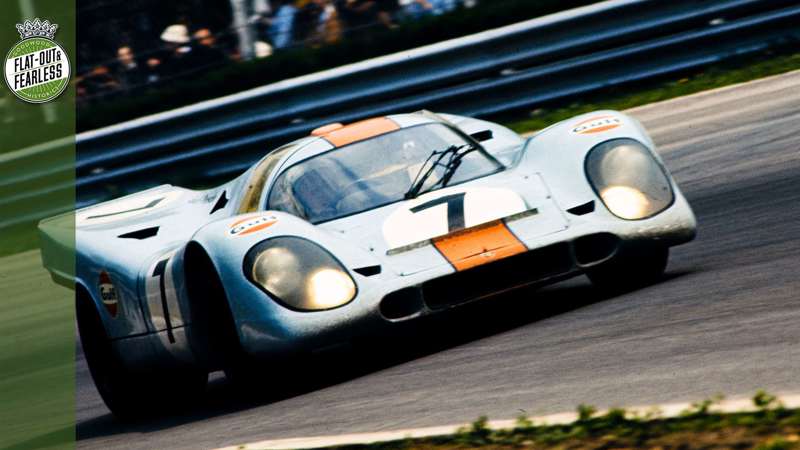This is a detailed photograph of a sleek, low-to-the-ground race car in the middle of a race on an outdoor racetrack. The car features a wide body with pointed and rounded lines at the front, adorned with large headlights and a dome-like cockpit where the driver sits. The vehicle exhibits a distinctive light blue design with an orange stripe running down the front, accompanied by the number seven prominently displayed on the hood and side panels within white circles. Additionally, the iconic Gulf Oil logo can be seen on the car.

The racetrack is elevated with a silver top rail and three lower blue rails surrounding the perimeter. In the upper left corner of the image, there is a green text area featuring a circular logo with the inscription "Flat-Out and Fearless," crowned with an illustrated crown. Within the logo, the text “Goodwood” and “Weston CT” are visible, emphasizing its association with the prestigious Goodwood racing events.

The sun is situated behind the car, casting a bright reflection that enhances the visual appeal of the scene. In the lower right portion of the image, a glimpse of the grass lining the inside of the track can be seen, adding to the outdoor ambiance of the location. The car's headlights are on, illustrating it in motion as it navigates the intricate curves of the racetrack.